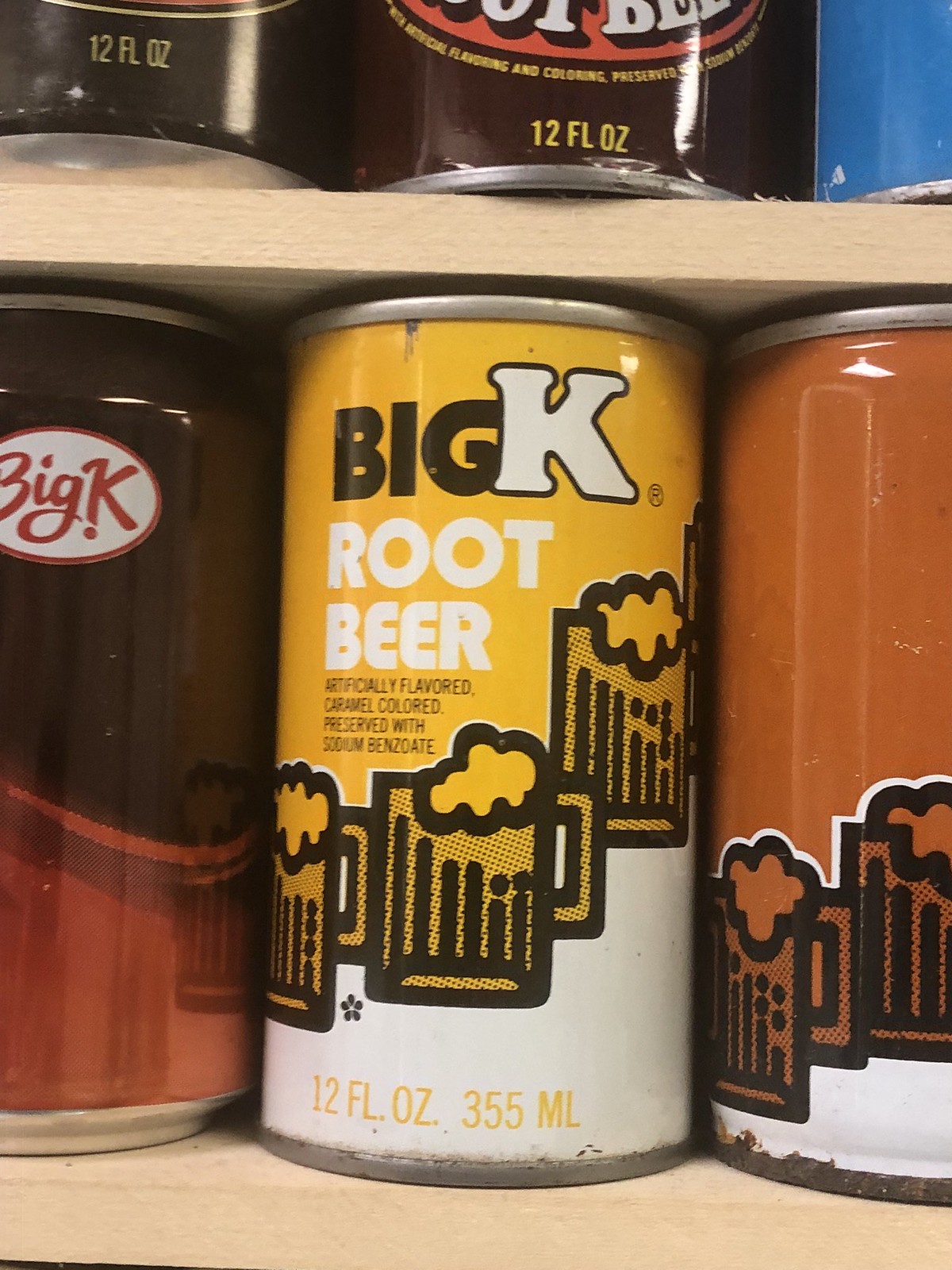This photograph shows a close-up view of two pantry shelves, displaying several root beer cans with various designs. The light unstained wooden shelves, just as tall as the cans themselves, house a collection of Big K root beer cans prominently positioned. The focal point of the image is a can labeled "Big K Root Beer," featuring a mustard yellow top and a white bottom, adorned with diagonal clipart drawings of mugs filled with foaming root beer. To the left, another Big K can is brown at the top with a lighter brown bottom, displaying the logo within a white oval. To the right of the focal can, there is a similarly designed can, but in brown and not yellow. The top shelf reveals partial views of three cans, two of which are brown and hint at root beer labeling, identifiable by segments of the text "O-T B-E" and "12 fluid ounces." A light blue can is also partially visible on the top right. The shelves provide a neat and organized display of nostalgic root beer beverages, emphasized by the classic and playful mug illustrations on the cans.